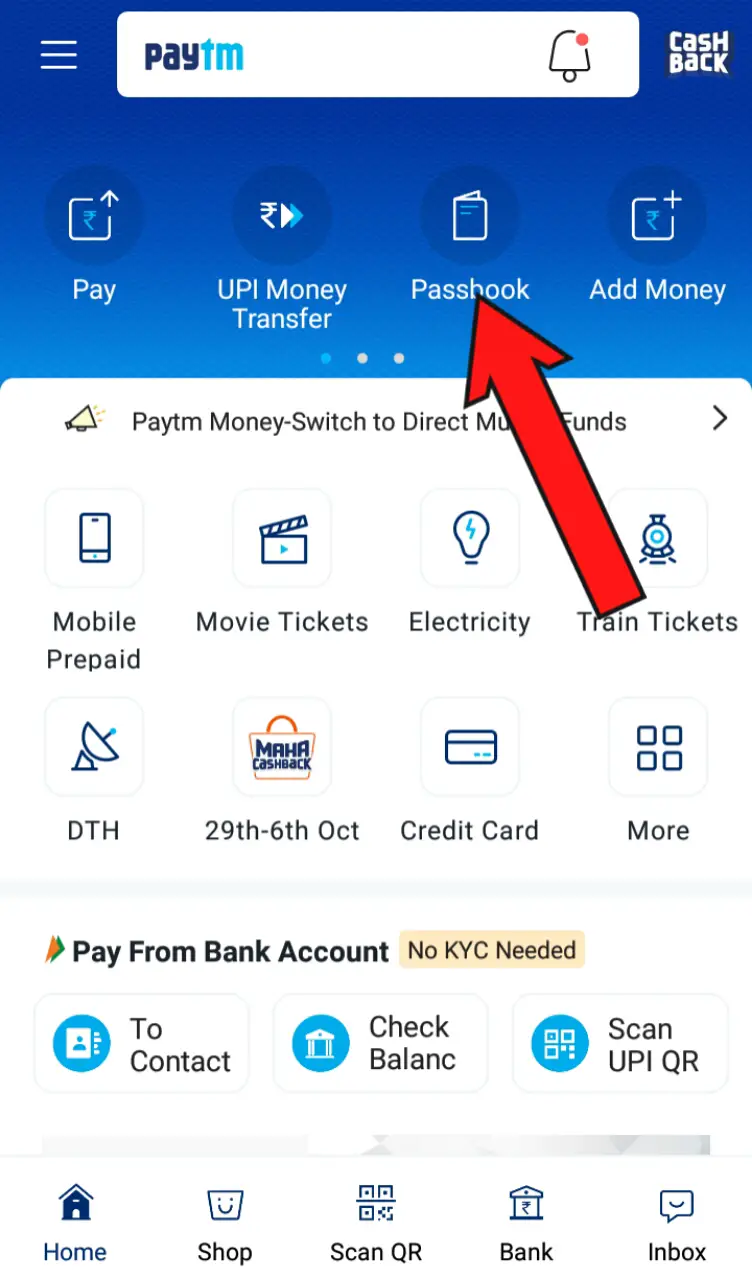This is a detailed screenshot of a mobile phone displaying the PayTM website. At the top of the screen is a purple header. In the upper left corner, there are three horizontal white bars, indicative of a menu icon. Next to the menu icon is a white rectangle with the text "PayTM," where "Pay" is in black and "TM" is in light blue. On the right side of this rectangle, there is a bell icon with a small red dot, likely indicating a notification, and to the far right, the word "Cashback" is displayed.

Below the header, there are three clickable buttons labeled "Pay," "UPI Money Transfer," and "Passbook." A bold red arrow has been photoshopped to point conspicuously at the "Passbook" button. Adjacent to these buttons is an "Add Money" option.

Beneath this section, against a white background, there is a text line: "PayTM Money: Switch to Direct Mutual Funds." Following this are two rows of four buttons each. The top row includes: "Mobile Prepaid," "Movie Tickets," "Electricity," and "Train Tickets." The bottom row contains: "DTH," a date marking "29-6 October," "Credit Card," and a "More" option.

At the very bottom of the screen, the text reads, "Pay from Bank Account."